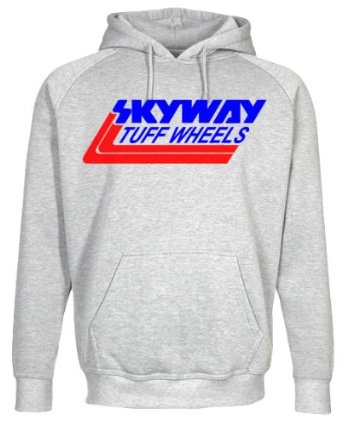The image features a light gray pullover hoodie with a soft, mottled gray and white texture. The hoodie has a large front kangaroo pocket and is equipped with long sleeves that end in cuffs, as well as cuffed waist. The hood is folded back, featuring short, basic gray drawstrings hanging down. At the chest level, there is a prominent logo. The logo includes a stylized red 'L' and sky blue text reading "Skyway Tough Wheels." The 'S' in "Skyway" is notably stylized with two red lines extending downward, bending and curving to incorporate the text, creating a dynamic design that runs parallel to the "Tough Wheels" text. The background of the image is white, emphasizing the details of the hoodie.